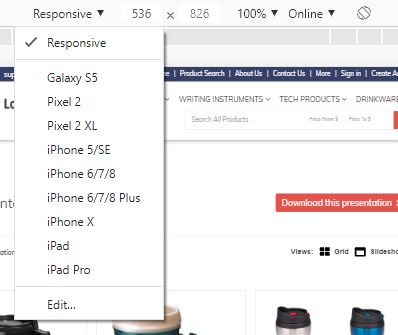A web page showcasing a responsive design is depicted. At the top of the page, there is a header labeled "Responsive" with a small triangular arrow beside it, indicating a clickable dropdown menu. When expanded, this menu reveals a list of device options including Galaxy X5, Pixel 2, Pixel 2 XL, iPhone 5/SE, iPhone 6/7/8, iPhone 6/7/8 Plus, iPhone X, iPad, and iPad Pro. Below this list, a slim gray line can be seen, followed by an "Edit" option accompanied by three dots.

Adjacent to this section, details include dimensions labeled as "536 x 816," a "100%" zoom level with a dropdown indicator, and an "Online" status represented by a black rectangle with a phone icon and directional arrows, hinting at the capability to change device orientation on the page.

Beneath these headers, an array of product images—appearing to be thermoses or water bottles—is displayed. Users are given options to view these products either in a grid layout or as a slideshow. An orange rectangle box labeled "Download this Presentation" provides an option to save the displayed content.